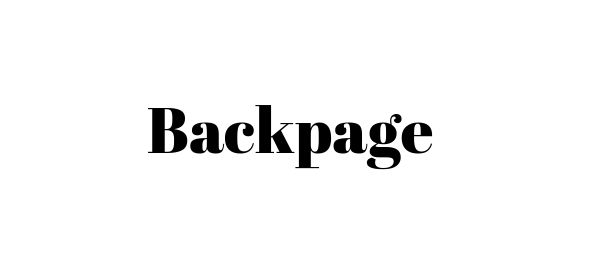The image features a solitary word, "Backpage," displayed in a striking, elegant font against a plain white background. The text "Backpage" is formatted as a single word with a capital "B" followed by lowercase letters. The font used exhibits a distinct design with varying thicknesses, transitioning smoothly from thin to thick strokes that give it a refined and artistic appearance.

The capital "B" has pronounced edges, extending slightly at the top left and bottom left corners, giving it a sturdy yet ornate look. The lowercase "a" starts with a dot at the top, curving gracefully downwards with a slight flourish at the bottom, reminiscent of a cursive style but still adhering to a standard font form. The "c" features a small circular flourish at its beginning, widening in the middle before tapering off again. 

The "k" is characterized by an extended line at the top of its upward stroke, adding an extra touch of detail. The "p" mirrors the decorative style of the "k" with lines accentuating both its top and bottom ends. The second "a" follows the same elegant style as the first. Finally, the "g" is noteworthy for its cursive-like, looped design with a small circle at the top, finishing with a delicate curl at the bottom.

Overall, the detailed and ornate font style of "Backpage" against the simple white background provides a sophisticated and visually engaging image.